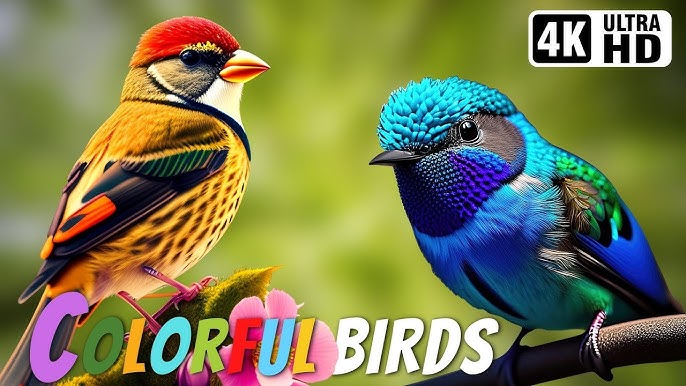The image showcases an advertisement on a 4K Ultra HD television screen, featuring two striking and vividly colorful birds against a blurry, green forest background. The headline at the bottom reads "Colorful Birds," with each letter of "Colorful" depicted in a different vibrant hue: C is lavender, O is green, L is yellow, O is light blue, R is lime green, F is red, U is light blue, and L is yellow, while "Birds" is in white.

The bird on the left is an exquisite blend of colors: it has a red mohawk-like crown, a golden-orange beak, and black eyes with surrounding regions painted in shades of yellow, black, and gray. Its throat and neck are white, transitioning into a tiger-patterned belly in shades of orange and black. Its wings are spectacular, flaunting a mix of blue, purple, orange, and green. It perches delicately on a green plant adorned with pink flowers.

The bird on the right is predominantly various shades of blue, with a light blue crown, a black beak, and black eyes highlighted by a green area. Its throat and belly exhibit different shades of blue, complemented by a black line, while the wings display an intricate mix of blue, green, white, and black. This bird's feet are black, and it is perched on a dark branch. The hyper-realism of the birds and their detailed portrayal underscores the television's high-definition capabilities, making for an eye-catching advertisement.